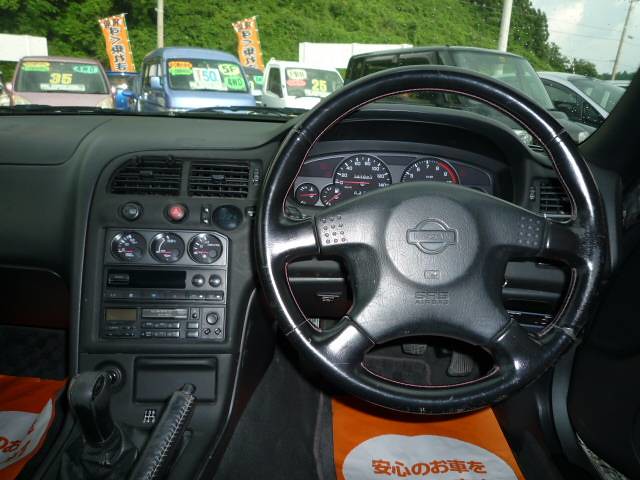The photograph captures the interior of a Nissan car taken from the driver's seat, showcasing a black leather-trimmed steering wheel with the Nissan logo. The dashboard and instrument cluster are predominantly black, with digital gauges and displays. Below the dashboard, the air conditioning panel, radio, and music system are visible, along with a gear stick and a handbrake lever. The floor features orange mats with Japanese writing. Through the windshield, an array of parked vehicles is visible, each marked with different numbers and stickers indicating they are for sale. Notably, a brown car with green and yellow decals bears the number 35, a light blue car is marked with 50, and a white car displays the number 25. Additionally, an orange banner with Japanese writing and a scenic green hill with trees can be seen in the background beyond the parked cars.